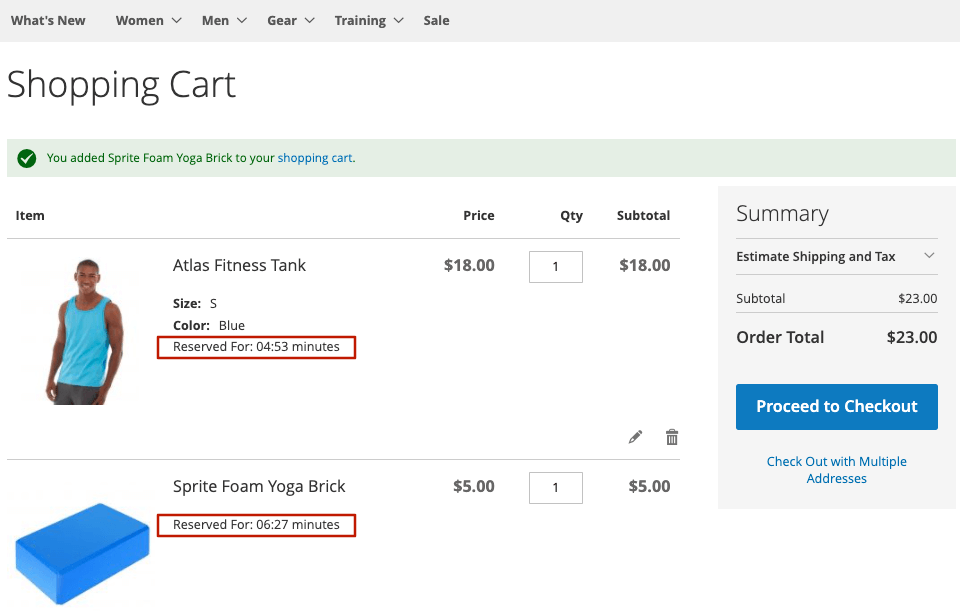In the described image, it appears to be a screenshot of an online shopping cart. At the top, there's a navigation bar featuring various sections such as "Grace," "What's New," "Women," "Men," "Gear," "Trading," "Sale," and a "Shopping Cart" icon. Below the navigation bar, there is a green checkmark indicating that an item has been added to the cart.

The shopping cart summary includes two items:
1. An "Atlas Fitness Tank" in blue, worn by a person who is also shown wearing gray shorts. The tank top is reserved for 4 hours and 3 minutes, priced at $18, with a quantity of 1, bringing the subtotal to $18.
2. A "Foam Yoga Brick" in blue, reserved for 6 hours and 27 minutes, priced at $5, with a quantity of 1, resulting in a subtotal of $5.

On the right side of the cart summary, there's a section labeled "Squares Summary" in black text, followed by "Estimate Shipping and Tax." The subtotal for the cart is listed as $23, the order total is also $23. There is a blue rectangle button labeled "Proceed to Checkout," alongside an option to "Check Out Multiple Addresses."

This comprehensive shopping cart contains a fitness tank top and a foam yoga brick.